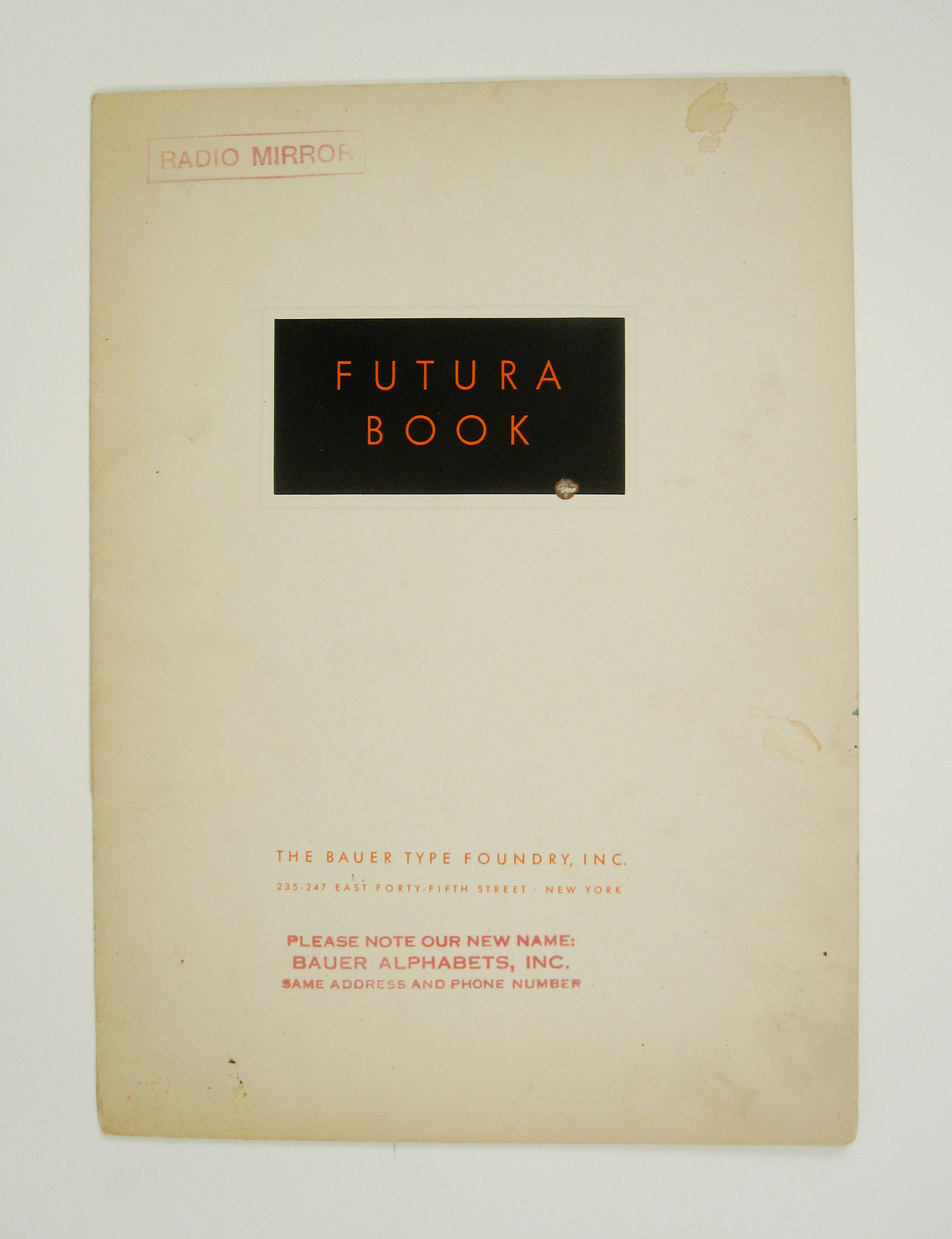This image depicts a broken link illustration, evidenced by the lack of visible objects or text. The graphic is characterized by an absence of discernible colors except those associated with the broken link symbol. This is prominently featured within a rectangular area, vertically aligned and off-white in hue. Superimposed in the middle is a book illustration with an off-white cover. On the upper left corner of the book is a light red rectangular stamp labeled "Radiomir." Centrally located at the top, a black rectangle with the red text "Futura Book" is visible. Below this, in a lighter red typeface, the text reads: "The Bauer Type Foundry, Inc., 235-247 East 45th Street, New York." Further down, another red stamp is noted with the message, "Please Note Our New Name, Bauer Alphabets, Inc., same address and phone number." Despite these intricate details, it's crucial to note that the actual image appears broken and is fundamentally inaccessible.